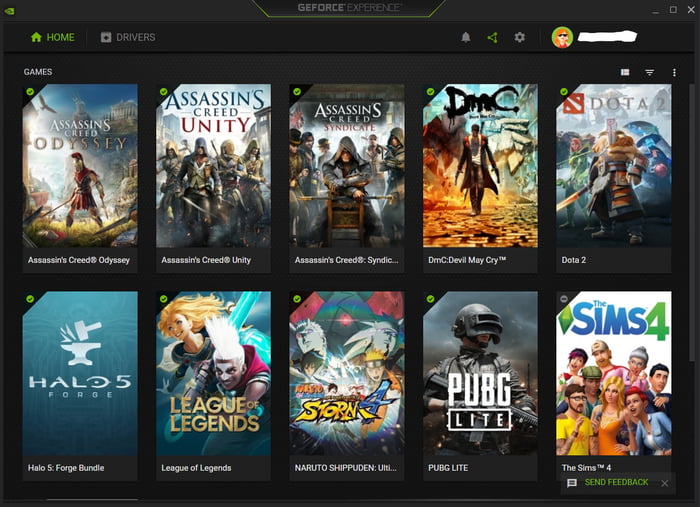The image appears to be a screenshot of someone's computer displaying a collection of video games. On the left side of the screen, a green "Home" button is visible, and to its right, there is an option labeled "Drivers." On the far right, there is a profile icon represented by a green bubble featuring an avatar of a red-haired individual wearing sunglasses, with the information next to it obscured.

The screen showcases two rows of video games. In the top row, starting from the left, is "Assassin's Creed Odyssey," which is represented by an image of a warrior wearing a helmet adorned with a red feather, a red skirt, and holding a sword. Next is "Assassin's Creed Unity," depicted with four fighters wielding swords. Following that is "Assassin's Creed Syndicate," which shows a figure in a gray cloak positioned centrally. The next game is "Devil May Cry" featuring a character in a long brown coat walking on what seems to be a golden path. The final game in the top row is "DOTA 2," illustrated by an armored individual brandishing a sword.

The bottom row starts with "Halo Forge Bundle," indicated by the text "Halo 5" and an image of an anvil and hammer. Next is "League of Legends," showing a female character with blonde hair and a male character with white hair. Then comes "Naruto Shippuden," featuring some animated characters. Finally, the row concludes with "PUBG Lite" and "Sims 4."